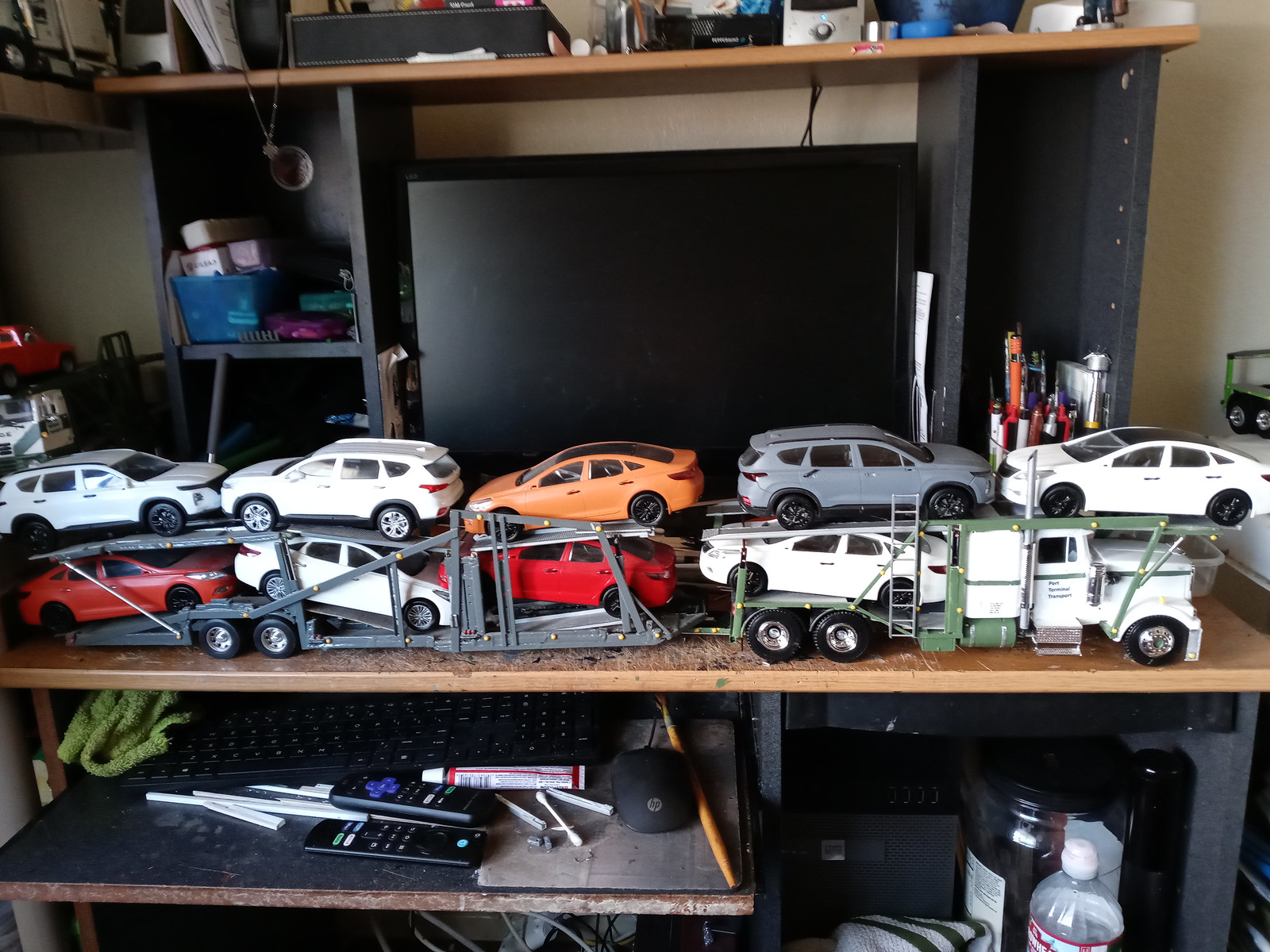The image depicts a cluttered interior of a house, focusing on a workbench that doubles as a computer desk. The most prominent feature is a worn brown shelf displaying an intricate toy car transporter truck. This truck, facing right, carries a variety of small model cars, arranged across two levels—four cars on the bottom and five on the top—each in different colors and orientations. Behind the truck is a black monitor, accompanied by several compartments.

The desk's surface below the shelf is strewn with miscellaneous items, giving it a messy appearance. A black keyboard, partially concealed by a green microfiber cloth, sits beneath the shelf. Nearby are various pens and pencils in different colors, a black Roku remote with multiple buttons, and a couple of unidentifiable black sticks, one labeled "HP." Additional clutter includes a dirty Q-tip, a tube with a white cap, and assorted random objects.

Above the main shelf, a higher, partially visible shelf holds even more disordered items, including a speaker, bottles, and bins, contributing to the overall cluttered ambiance.